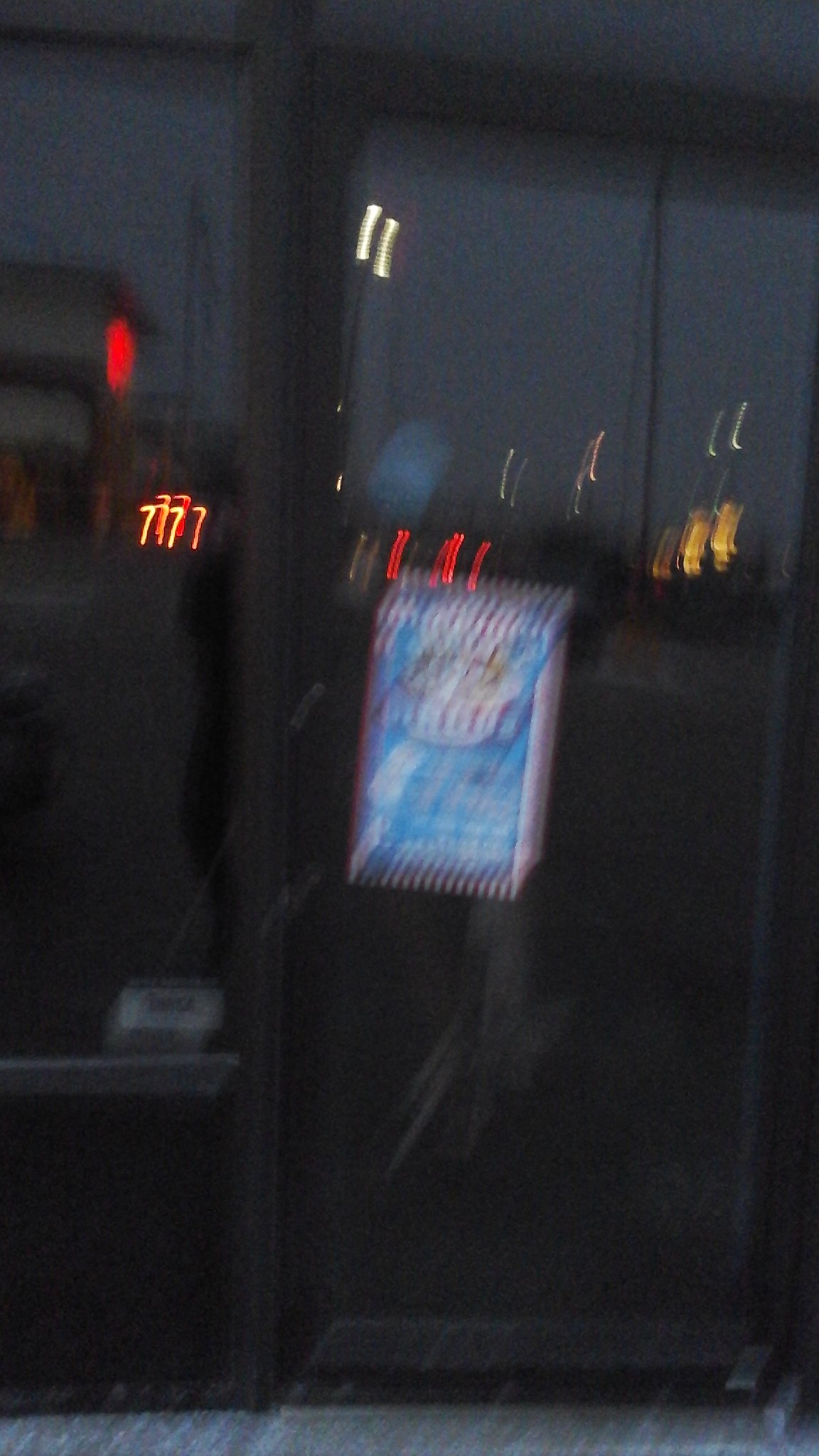This blurry, night-time photograph appears to capture a storefront with a glass door and a large window to its left. The image is in portrait format, suggesting it was likely taken with a mobile phone. Despite the heavy blur, several details are discernible. The window on the left features a section of the wall beneath it, which is black and about a foot high off the ground. Pavement is visible beneath this wall section. Reflections in the glass—including a building with a red light and an orange light below it—are apparent. The storefront's glass door has a blue, red, and white poster in the middle, though the text is unreadable. Additional reflections of various lights are scattered across the door and window, with recognizable colors including red, orange, white, and yellow, adding splashes of color to the scene. The dominant lights reflect the numbers "777" in neon yellow on the left and assorted flecks of color (white, red, and yellow) throughout the image. The overall blurriness leaves the specific context and exact details ambiguous, contributing to its enigmatic, almost abstract quality.